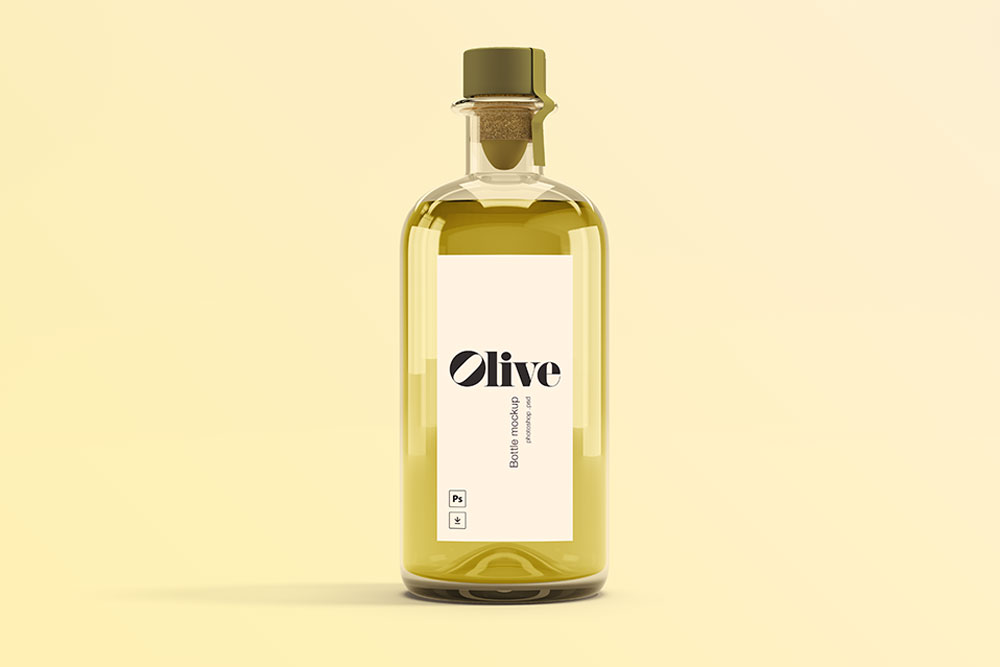An olive oil bottle sits gracefully on a tan background that subtly transitions into a pinkish hue towards the right. The bottle, reminiscent of an old-fashioned apothecary design, is made of glass and tapers into an olive green top with a matching cork stopper that gives it a rustic charm. The stopper is secured with olive-colored tape. Inside, the bottle is filled with a gold-hued liquid that nearly reaches the base of its neck.

Prominently displayed in the center of the bottle is a vertical white label with elegant black text. The label reads "Olive Bottle Mock-up," with "Olive" featuring an O tilted diagonally to the right in a stylized, 1970s script. Additionally, in the lower left corner of the label, framed by a thin black border, is a small box containing "P.S." and a downward-pointing arrow. This detailed and intricate design adds to the nostalgic feel of the bottle. The positioning of the bottle, centered against its warm background, suggests a setting either in a household environment or on display in a store, perhaps hinting at its versatile use as either a culinary ingredient or a skincare product.